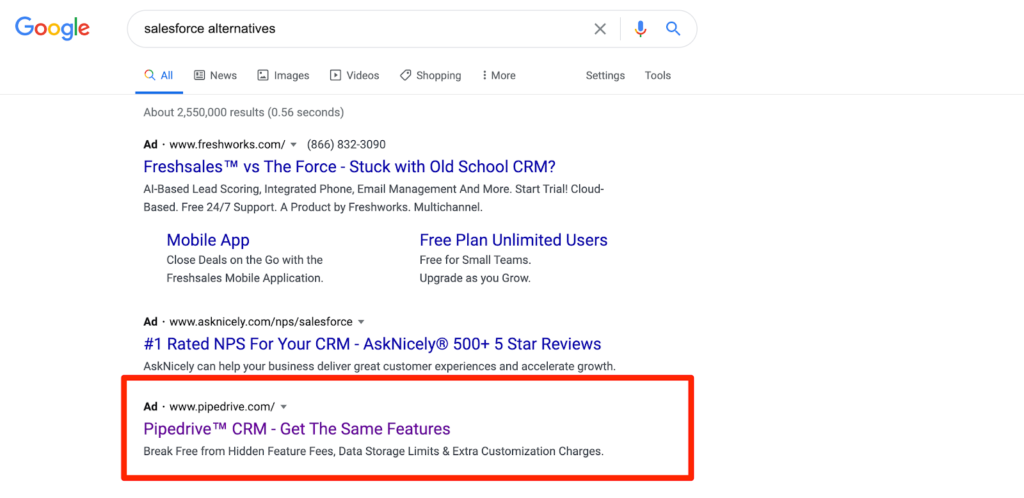Here is a cleaned-up and detailed caption for the described screenshot:

"A Google search screenshot shows a query for 'Salesforce alternatives' on a white background. The colorful Google logo (blue, red, yellow, blue, green, red) is displayed in the upper left corner. Within the search bar, the query is visible alongside an 'X' to clear the text, a microphone icon for voice search, and a magnifying glass icon for initiating the search. Below the search bar, navigation options are listed, including All, News, Images, Videos, Shopping, More, Settings, and Tools, with 'All' currently selected. The search results indicate there are approximately 2,555,000 results found in 0.56 seconds.
   
Highlighted ads are displayed first. The first ad is from Freshworks (www.freshworks.com, (866) 832-3090) promoting 'Freshsales' as an alternative to Salesforce, featuring a mobile app, a free plan, and unlimited users. The second ad from Askniceway (www.askniceway.com) emphasizes its number-one rated NPS for CRM, citing over 500 five-star reviews and the ability to help businesses deliver excellent customer experiences and accelerate growth. The final ad from Pipedrive (www.pipedrive.com), marked with a red rectangular box and an ad logo, promotes 'Pipedrive CRM,' highlighting the same features as Salesforce but without hidden fees, data storage limits, and extra customization charges."